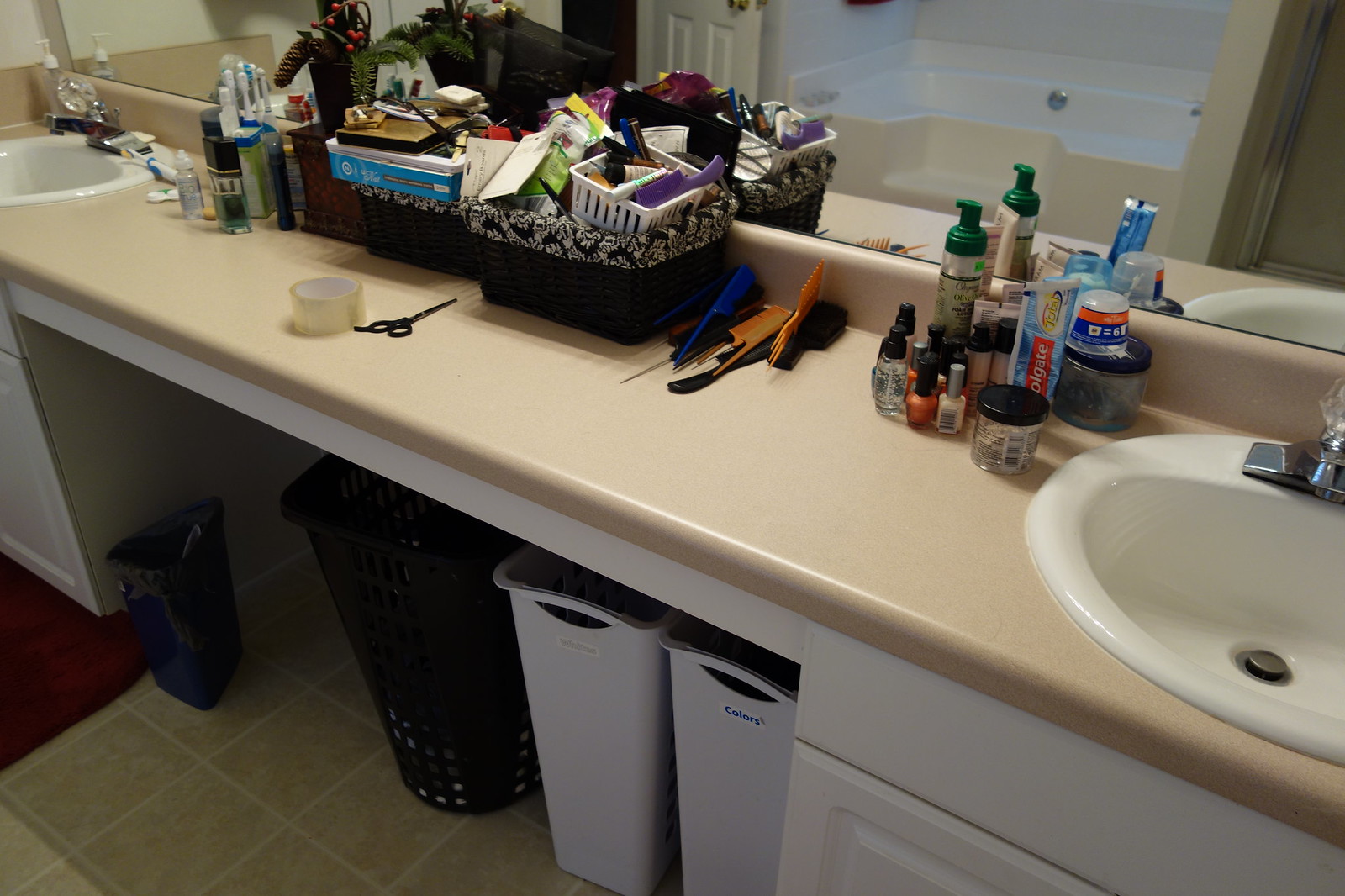This amateur photograph captures a cluttered bathroom counter in an upscale home. The counter features two white sinks separated by a wide stretch of beige countertop, above which hangs a mirror that reflects a spa-style tub and a shower situated at the back of the bathroom. An open door is visible in the reflection, adding a sense of depth to the scene. Below the counter are three laundry baskets, labeled "colors," and a smaller blue wastebasket lined with a black trash bag. The counter is crowded with everyday bathroom items, including toothpaste, grooming products, hair products, nail polish, and combs and brushes, suggesting the space is used frequently, possibly by someone who takes their grooming seriously.

Despite attempts to organize the clutter, with some items stacked in two black woven baskets with black and white fabric linings, there is still an overflow, giving the area a somewhat chaotic appearance. The floor is covered in beige tile with white grout, and a red bath mat is placed in front of one of the white sinks. The fixtures throughout the bathroom, including the tub, sinks, and cabinets, are white with chrome accents, adding to the overall clean and neutral aesthetic of the space. There's no text except for logos and packaging on the items, adding to the personal, lived-in feel of the bathroom.